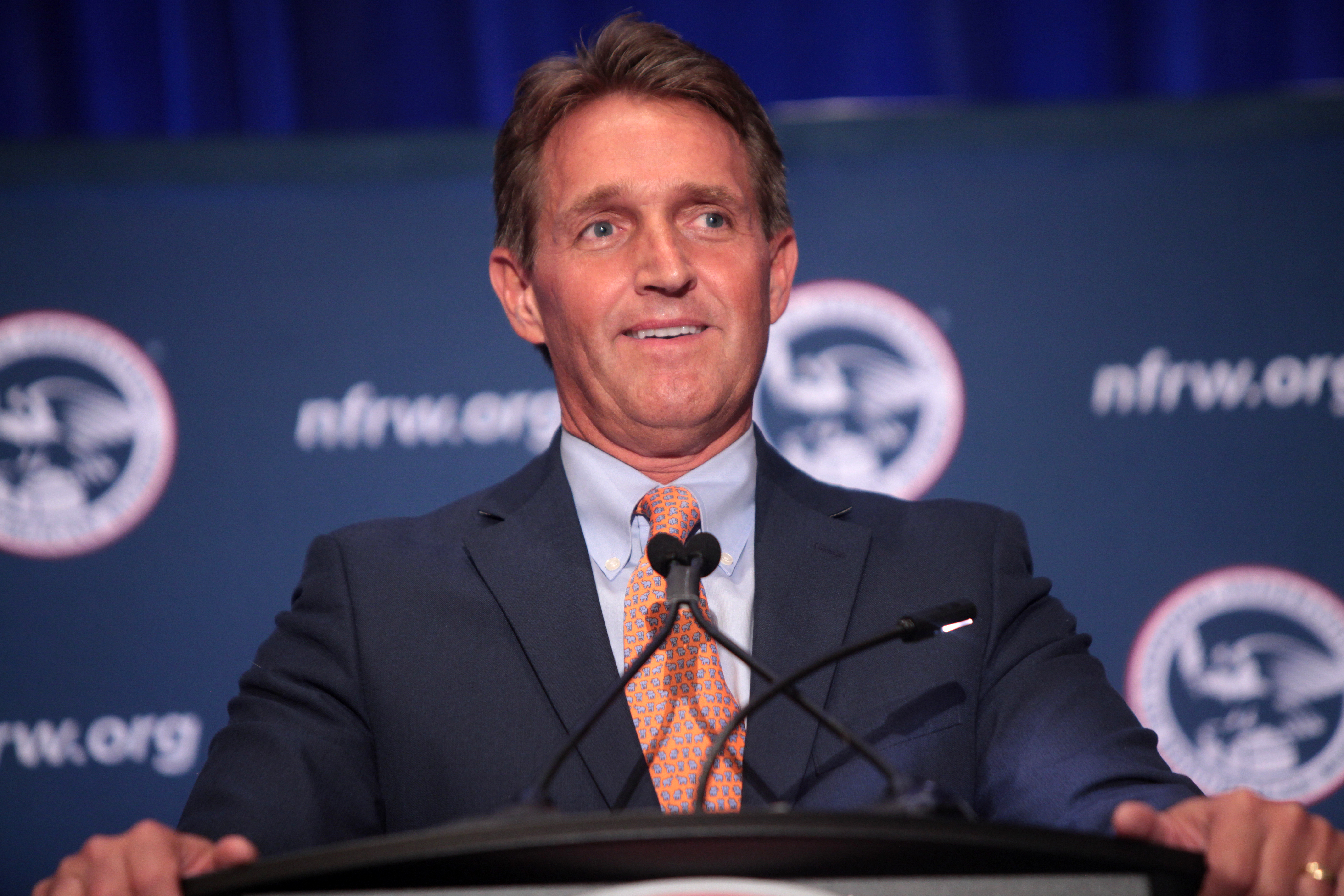A photograph captures a middle-aged white man, likely in his late 40s or early 50s, standing behind a black podium with an adjustable reading light that is currently on. The podium features a double-necked microphone, both ends pointing towards the man, who has his hands resting on it, revealing a ring on his left ring finger. The man, dressed in a dark blue business coat, a light blue button-up shirt, and a peach-colored tie with blue-gray dots, has light brown hair and appears to be looking slightly off to the right, with a subtle, amused smile on his face. Behind him, there is a large blue backdrop adorned with multiple white logos, including one that reads "NFRW.org" and another circular design with a red border. The background is slightly out of focus, keeping the emphasis on the man and the podium in the forefront of the image.